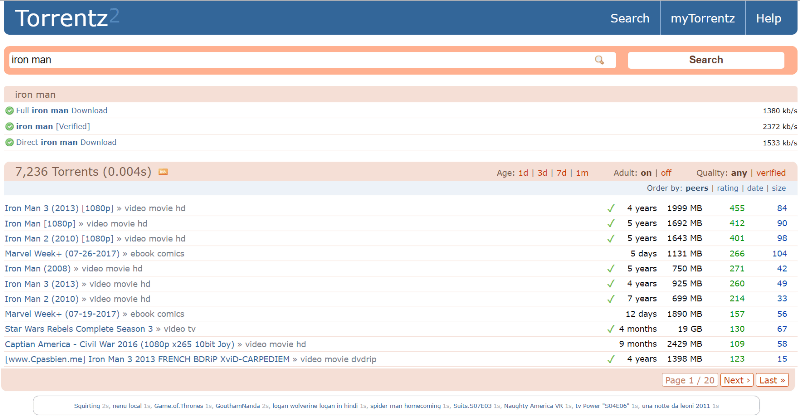At the top of the image is a dark blue box with the word "torrents" displayed prominently in white text, stylized as "T-O-R-R-E-N-T-Z". On the right side of this box, there are options labeled "Search My Torrents" and "Help."

Below this top box, a search bar bordered in pink is visible, featuring the placeholder text "Iron Man." To the right of the search bar is a button labeled "Search."

Under the search bar, there is a pink box containing the text "Iron Man." Beneath this, several options are listed: "Whole Iron Man download," "Iron Man [Verified]," and "Direct Iron Man download." Each option is accompanied by a green circle with a check mark in its center on the left side.

Lower on the page, another pink box displays the text "7236 torrents, 0.004s." Below this box, there's a list of time frames that include "Age: 1 day," "3 days," "7 days," and "1 month."

At the bottom, there's a final entry stating "Iron Man 3 (2013) 1080p Video Movie HD."